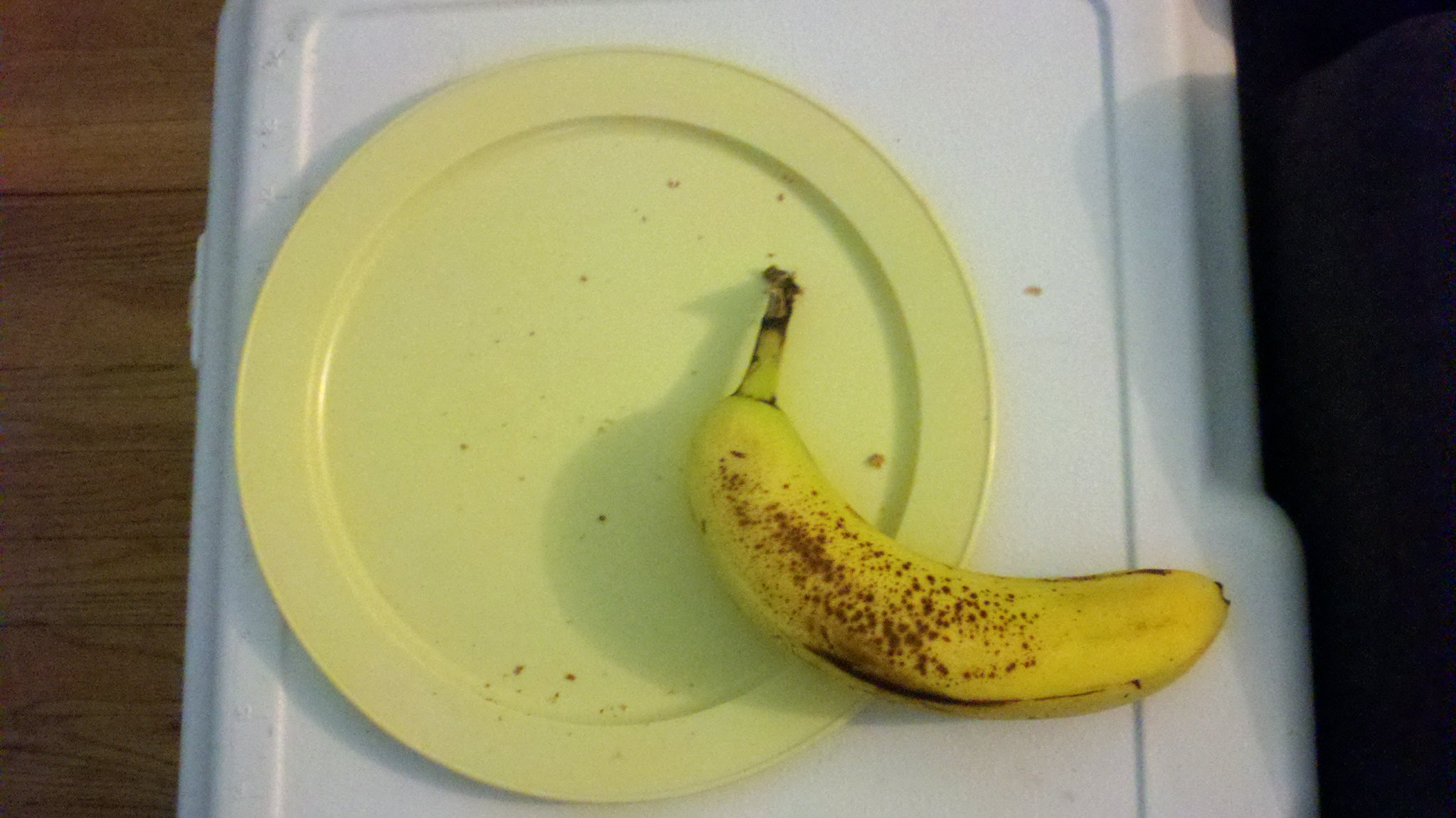In the image, there is a white plastic cooler positioned on a wooden floor, although the floor is more prominently visible on the left side of the picture due to better lighting, while the right side is obscured by shadows. The cooler's lid is clearly discernible, and part of a hinge is visible on the left edge, indicating it is designed to lift open. On top of the cooler, there is a yellow plate with crumbs scattered on its surface and one crumb having fallen onto the cooler lid. Also on the plate is an unpeeled banana, which is partly hanging off the edge. The banana has small brown speckles, suggesting it is ripening but not yet overly soft. There is a faint cast shadow to the right, possibly from a table with a lamp, suggesting that a light source is positioned nearby. The image's framing cuts off both the top and bottom edges of the cooler.